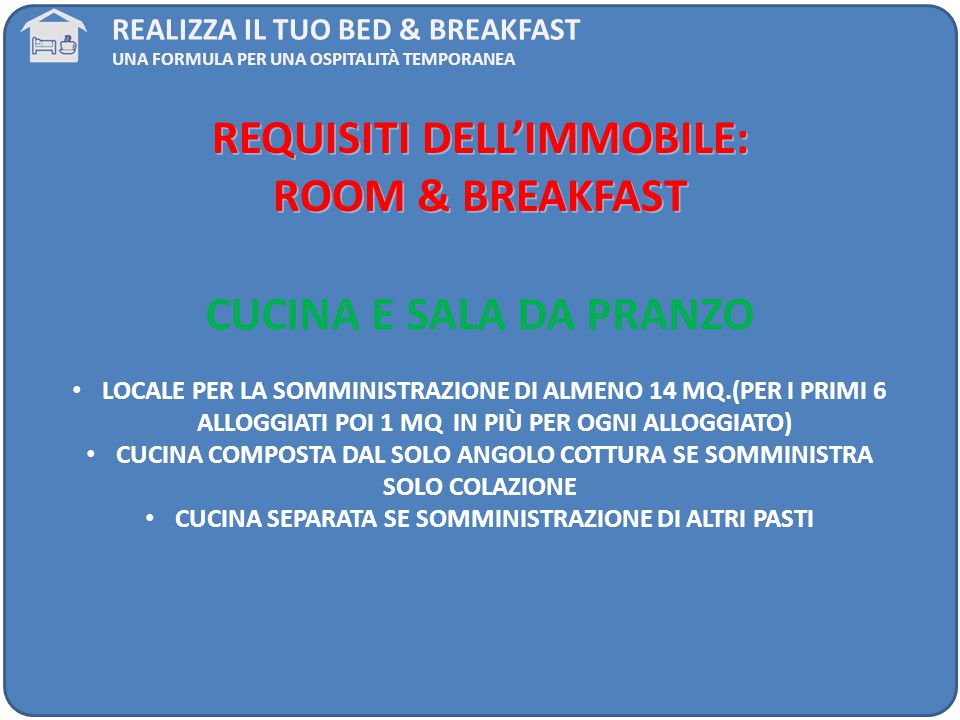This image appears to be an informational screen, likely from a website or a slideshow, detailing a bed-and-breakfast service. The layout is a wide, vertical rectangle with a solid blue background and rounded edges. In the top left corner, there is a small icon of a house with a bed, a coffee mug, and possibly a TV inside. 

To the right of this icon, in white text, it reads "Realizza il tuo bed and breakfast," followed by "una formula per una ospitalità temporanea." This content is in Italian. 

Centered in the upper portion of the screen, in red uppercase letters, the text reads "REQUISITI DELL'IMMOBILE: room and breakfast." A few lines below, in green uppercase letters, it states "CUCINA E SALA DA PRANZO." Below this green heading, there are three white bullet points containing additional white text that continue the description, all in Italian. The alternating colors of the text—red, green, and white—are consistent throughout the image.